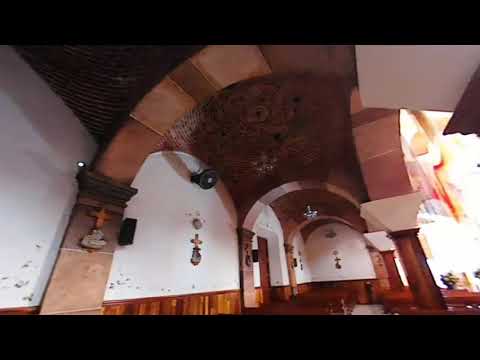The image depicts the interior of an old building, likely a church. The photograph is vertical and rectangular, framed by horizontal black lines at the top and bottom. The perspective is slightly upward, directing focus towards the ceiling. The ceiling is crafted in dark brown wood with an arched dome design, supported by large stone archways and brown columns. The walls are smooth, white concrete, adorned with multiple wooden crosses. Below, the walls are lined with brown wood paneling that extends about two feet from the floor. On the foreground left wall, an arched support column extends gracefully upwards and integrates into the ceiling. Adjacent to this, there is a cross mounted on the column and another on the white wall. Farther along the left wall, there are more crosses and an entryway. To the right side of the image, there is an indistinct area with some orange hues and possibly objects resting on a surface. This architectural and decorative detailing underlines the church-like solemnity of the space.